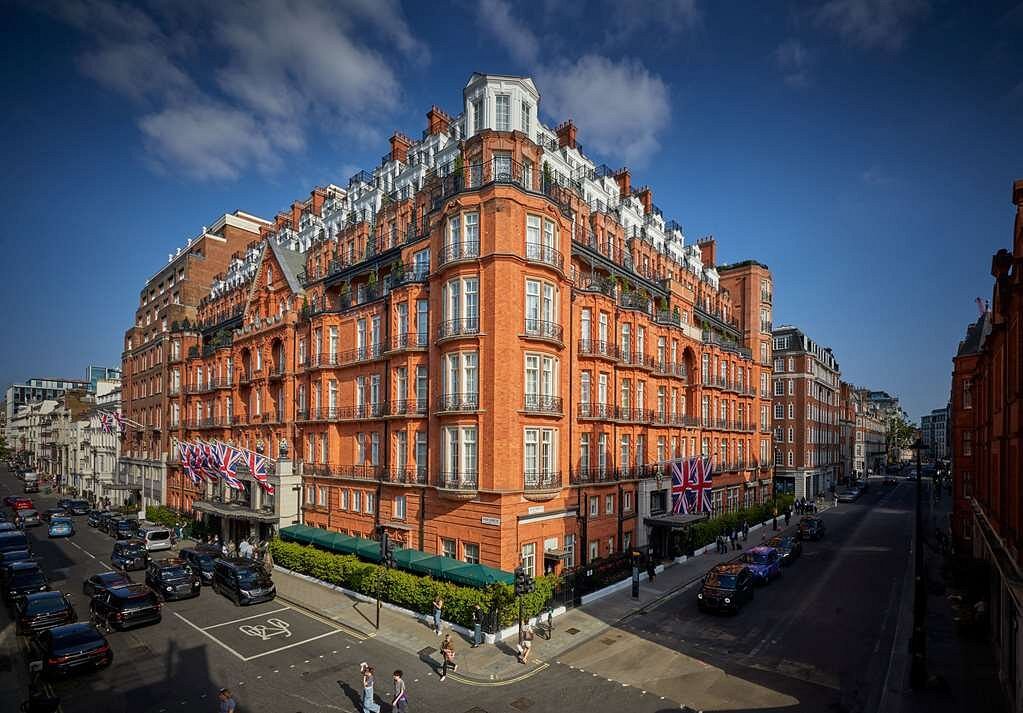This daytime photograph features an extremely large terracotta orange building adorned with numerous white-framed windows. The top portion of the building is painted white, contrasting with its primarily terracotta color. Black metal balconies are visible near the roofline. On the sides of the building, several Union Jack flags in shades of red, blue, and white are prominently displayed. In the foreground, green shrubbery and green awnings add a touch of nature to the urban setting. The background showcases additional buildings, some painted white and others in varying shades of terracotta. Two streets intersect near the building, bustling with people, a mix of darker and lighter colored cars, and a bicycle icon painted on one of the streets. The scene is set under a blue sky dotted with fluffy white clouds.